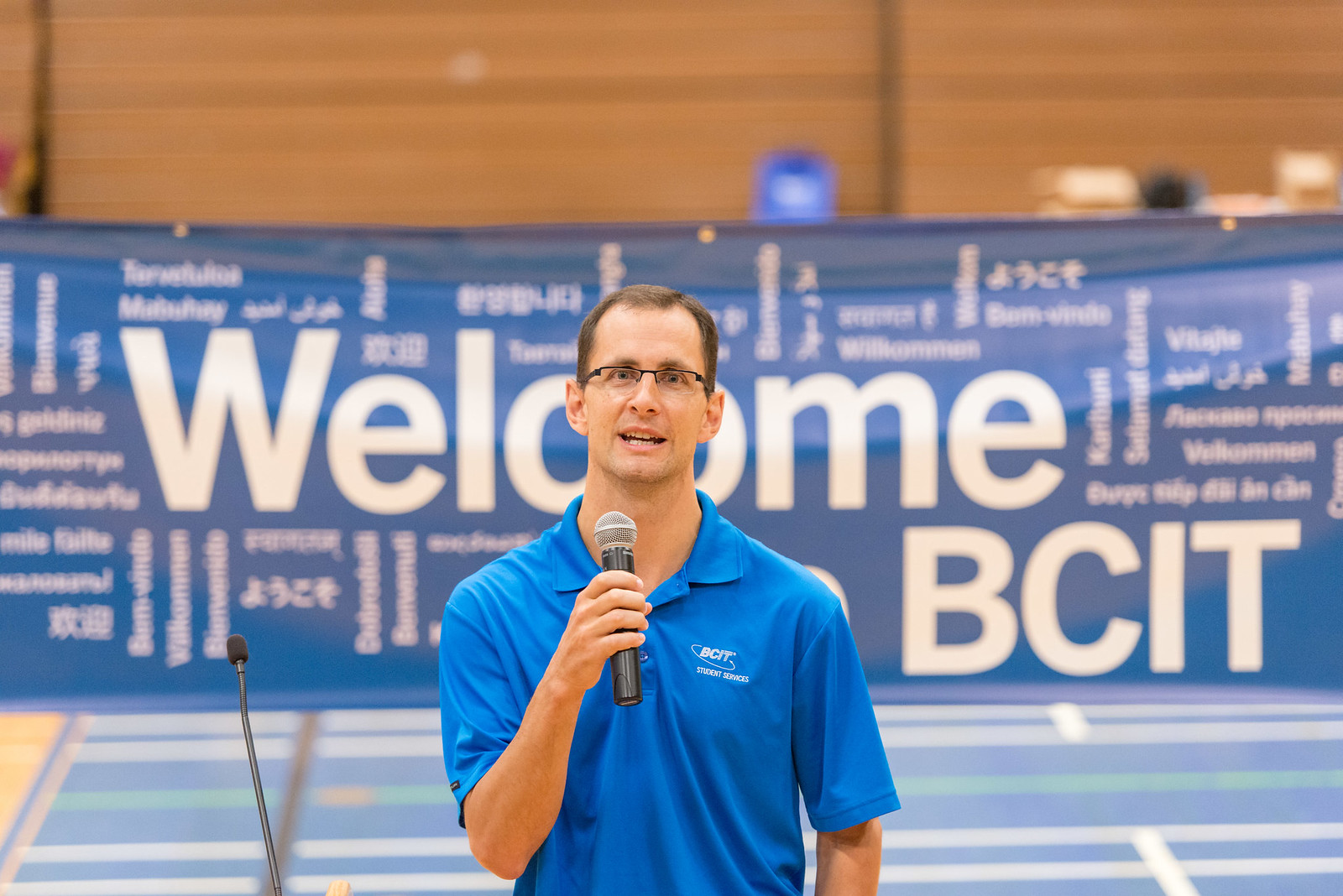A landscape-oriented color photograph captures a man centered in the frame, holding a microphone in his right hand and looking directly at the camera with a slight upward gaze. He has wire-rimmed glasses, short brown hair, and is wearing a blue collared shirt with a white emblem that reads "BCIT," matching the blue tones in the background and floor. The room resembles a gymnasium or an open convention space, evidenced by the blue floor with white stripes and markings. Behind the man, a large blue advertisement banner prominently displays the text "Welcome BCIT" in large, bold white letters, surrounded by smaller, illegible text in various directions and languages. The backdrop also includes what appears to be padded gymnasium walls in brown with horizontal stripes, adding to the venue's athletic or convergent setting. The man appears to be making an announcement, projecting a happy demeanor while engaging with the camera.